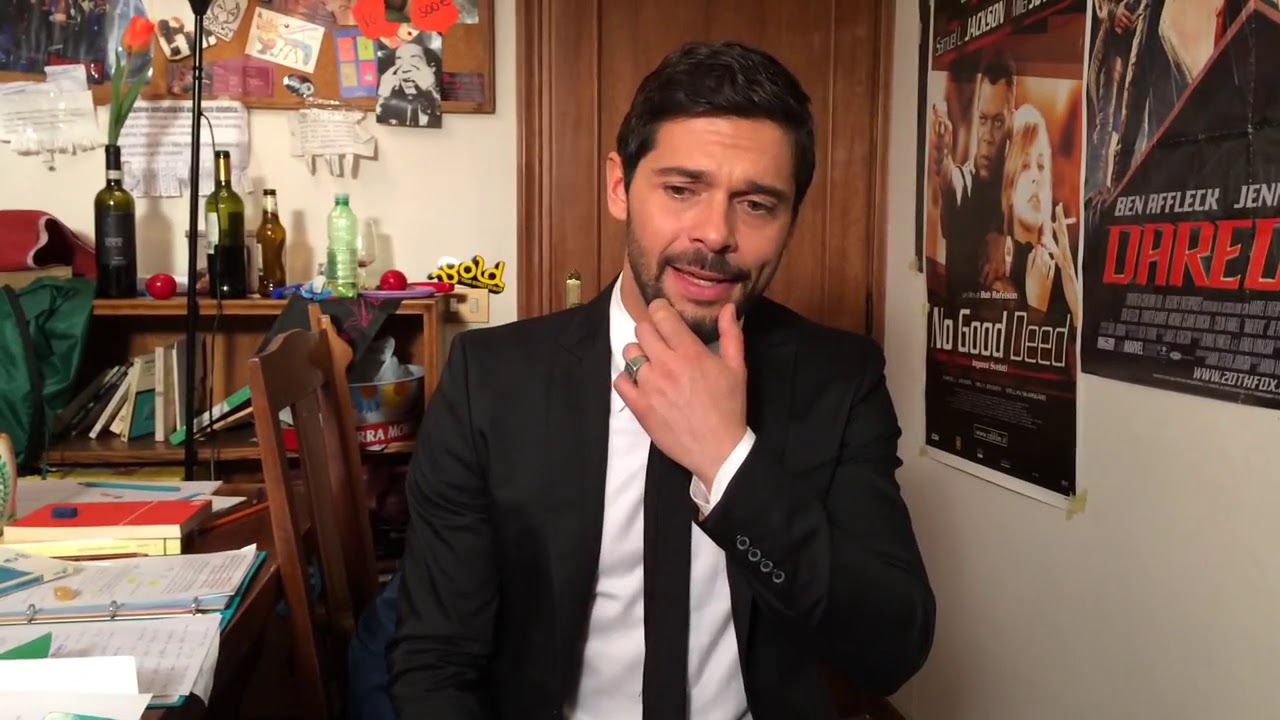A contemplative man with dark brown hair, a mustache, and a beard is seated sideways on a chair, facing the camera. He is dressed in a formal black suit, white dress shirt, and a black tie, with a ring visible on his left hand as he scratches his chin. The room around him is cluttered; to his left, there is a wooden table strewn with papers, books, a pen, and an eraser. Bottles, which appear to be wine and water bottles, are also scattered on the table. In the background, a corkboard filled with photos and random items is prominently displayed above a shelf lined with additional books and bottles. Directly behind him, a brown door is visible. To the right of the door, hanging on the wall, are two black and white movie posters: one reads "No Good Deed" featuring a black man and a white woman, and the other includes the names "Ben Affleck" and "Jen" with partially visible text beginning with "Dare."